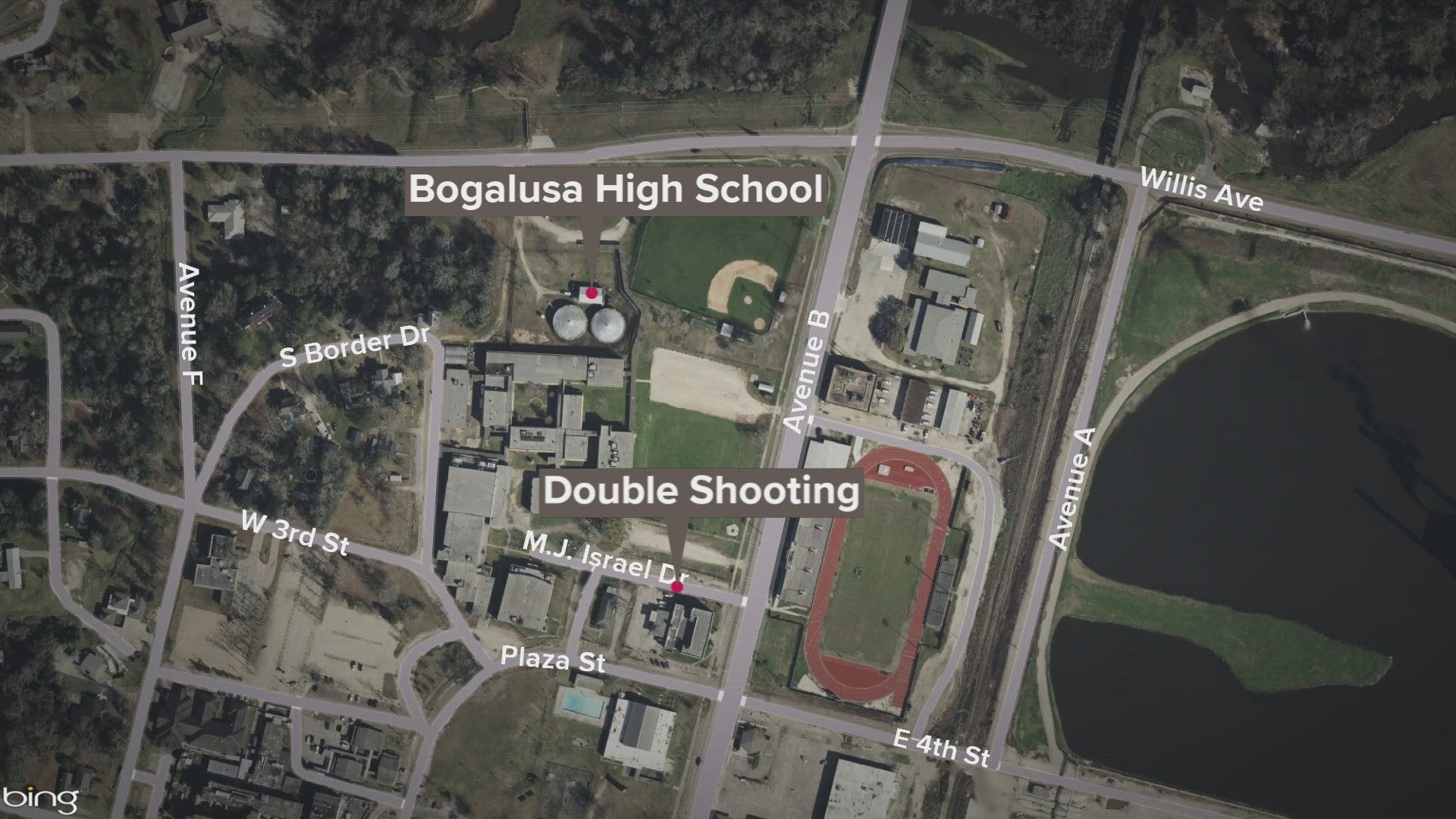This aerial satellite image of Bogalusa High School, sourced from Bing as indicated in the bottom left corner, provides a detailed view of the school's layout and surrounding area. The high school buildings, football field, and track are clearly visible. To the west of the campus, a large, man-made lake is evident with a road encircling it. Major roads such as Willis Avenue, East 4th Street, Avenue A, Plaza Street, West 3rd Street, South Border Street, and Avenue F are labeled, forming a grid around the school. The photograph prominently highlights a double shooting location on MJ Israel Drive with an arrow pointing to a red dot. Adjacent to the high school are various other sporting fields, including a baseball field. The comprehensive labeling of roads and the clear indication of the shooting incident make this a detailed and informative aerial view of the area.